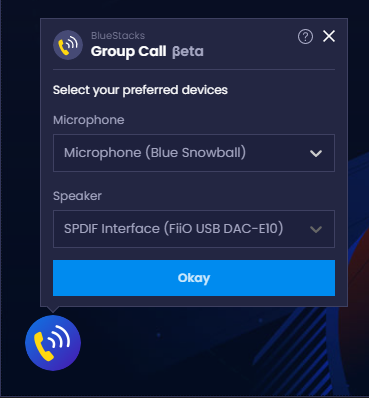The image depicts a screenshot of an application interface, captured in portrait orientation. The background is predominantly black with subtle blue accents, featuring intricate patterns that are difficult to describe. At the center of the image, a blue square with a blue background stands out.

At the top of this square is a lighter blue circle encompassing a yellow dot, from which a white signal-like icon emanates. Above this, the word "BlueStacks" is displayed in bold white letters, with the word "Group" next to it, followed by "Beta" in gray text. To the right, there is a question mark icon and a white 'X', all separated by a gray border.

Below this header, the text "Select your preferred devices" appears in white. The interface then lists "Microphone" in gray font within a blue box, specifically showing "Microphone: Blue Snowball" accompanied by a downward caret for additional options. 

Underneath the microphone selection, there is a speaker option labeled "S/PDIF Interface (FIIO USB DAC-E10)" with another dropdown caret for further selection. 

At the bottom of the interface, a light blue, clickable box with the word "OK" in white font is present. Beneath this button, there is an icon featuring a phone in a light blue circle, with an orange phone icon and a white signal emanating from it.